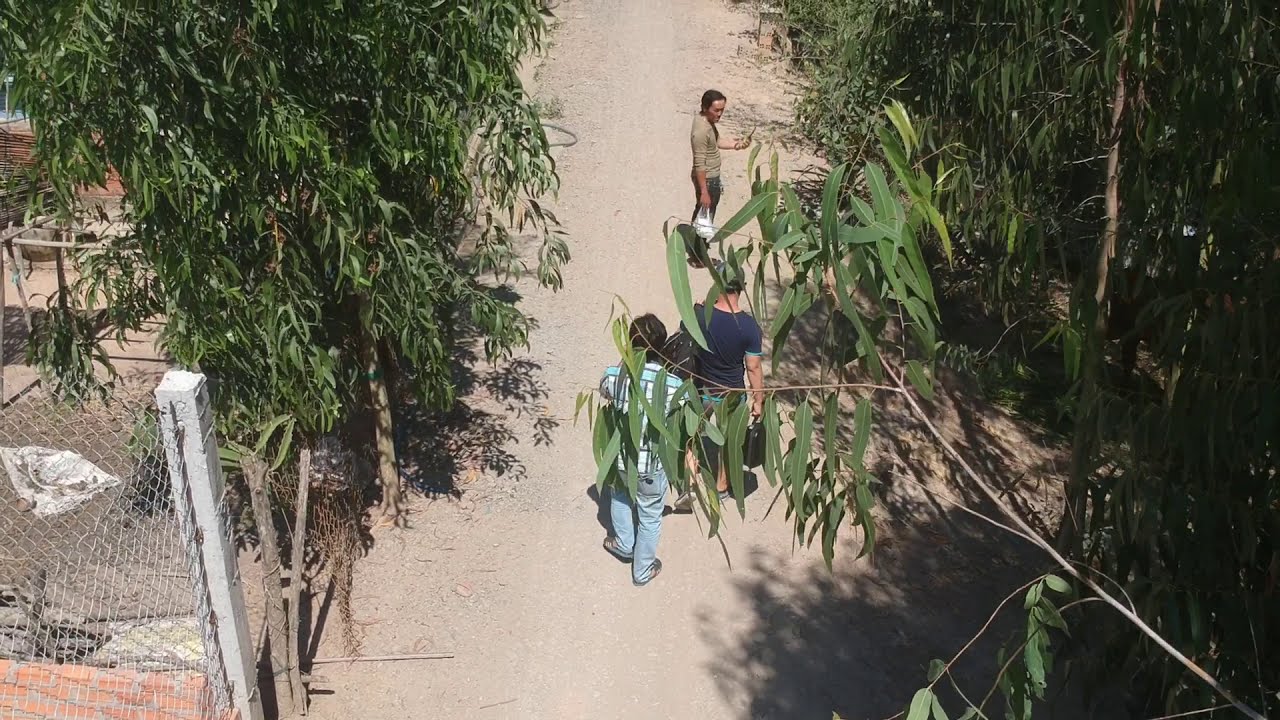In this detailed and vibrant overhead daytime photograph, likely captured by a drone or from an elevated position, three individuals are standing on a dirt walkway or road surrounded by lush, leafy vegetation, including tall bamboo trees. The image is in a landscape orientation with excellent clarity, showcasing natural light illuminating the scene. Two individuals, with their backs to the camera, appear engaged with the third person, who stands sideways, looking back at them while holding a white object in his right hand. The individuals are wearing variously colored clothing: one in a beige shirt with dark pants, another in a dark black shirt with obscured pants due to a leafy branch, and the third in a white and blue shirt with light blue jeans. The pathway is flanked by dense greenery on both sides, and at the bottom left corner, a partially visible white chain-link fence hints at a structured area, possibly suggesting a zoo or a park setting. Shadows from the bamboo add contrast and depth to the scene, enhancing its realistic representational style.